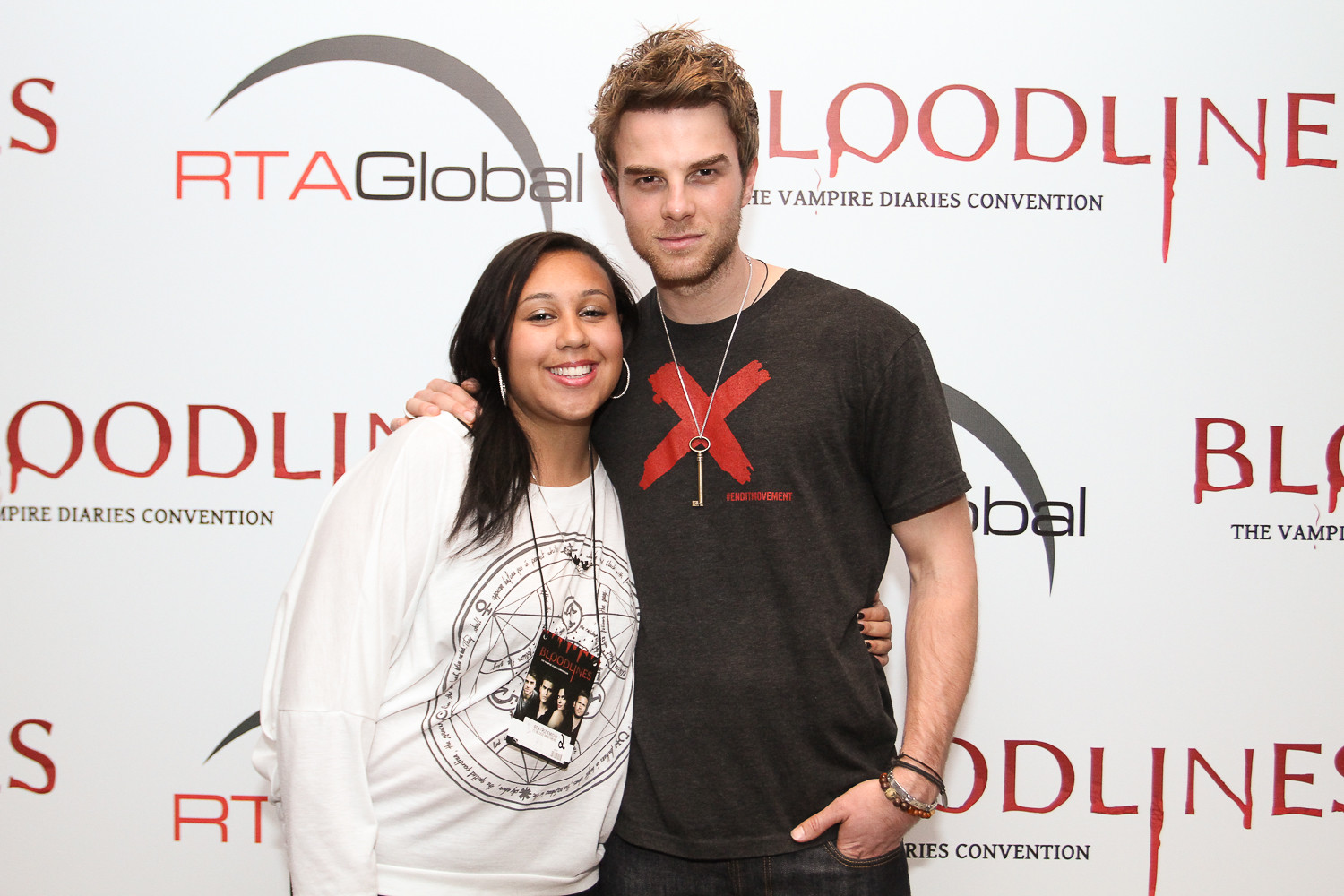The photograph features a young white male and a black female standing together, smiling at a "Bloodline: The Vampire Diaries Convention." The backdrop displays a white wall with "Bloodline" written in a drippy red font and "The Vampire Diaries Convention" in black. Additionally, there is a logo reading "RTA Global" in red and black, flanked by an abstract crescent shape.

The man, positioned on the right, has stubble and wavy brownish-blonde hair. He is wearing a black t-shirt with a prominent red "X" across the chest, dark jeans, a key necklace, and several bracelets. His left hand is in his pocket while his right arm is warmly wrapped around the woman’s shoulder.

The woman has straight black hair, hoop earrings, and is adorned with glittery eyeshadow and pink lipstick. She wears a white long-sleeve top featuring a black geometric design and a pass with images of four people on a lanyard around her neck. Her arm encircles the man’s waist. Both appear delighted, suggesting the woman is likely a fan posing with a celebrity at the convention.